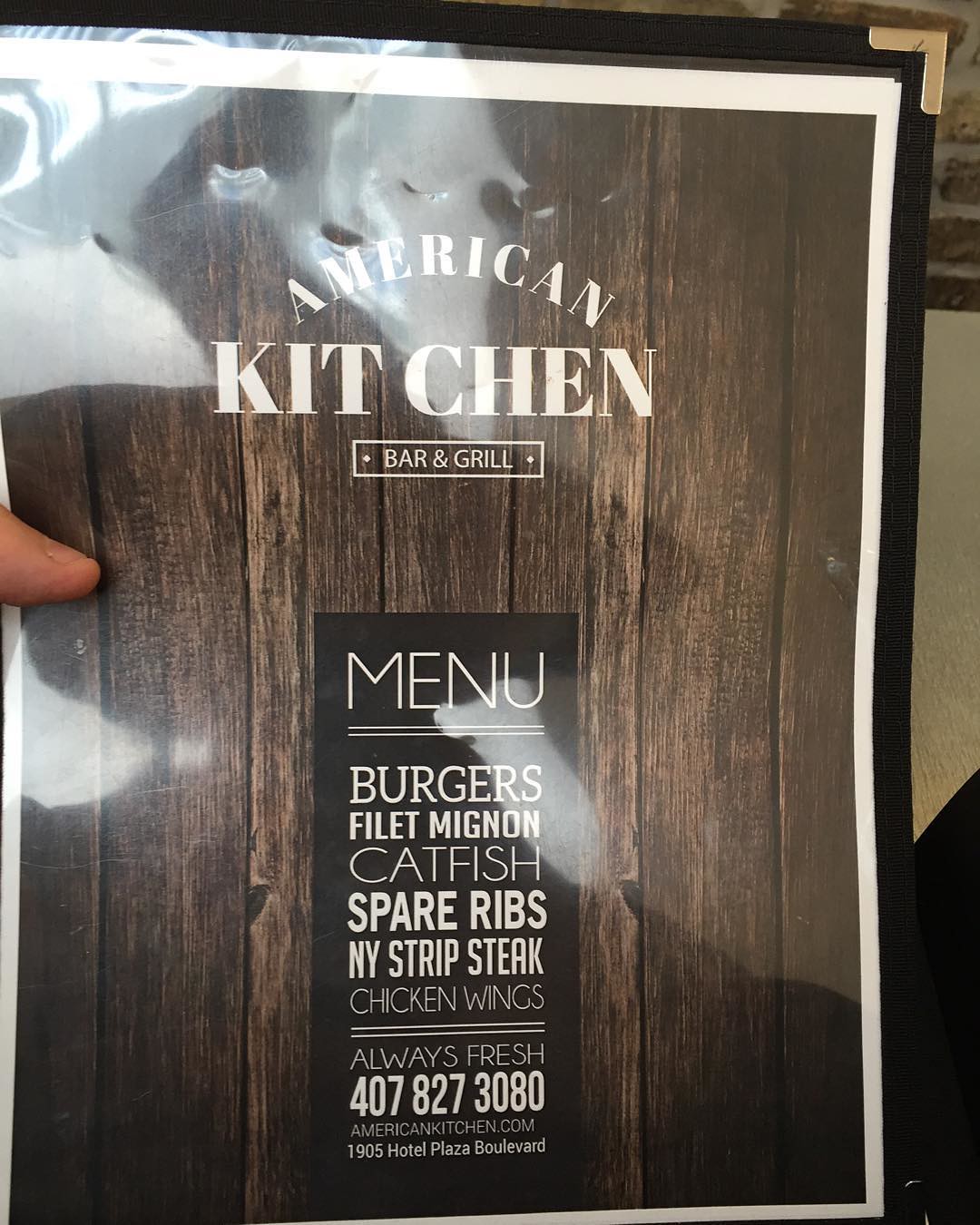An up-close photograph captures a menu from the restaurant, American Kitchen Bar and Grill. Dominating the center of the menu is the word "MENU" in large, bold letters. Below, a list of popular dishes includes burgers, filet mignon, catfish, spare ribs, New York strip, and chicken wings. Two lines underline these offerings, emphasizing the phrase "Always Fresh."

Further down, the contact information is clearly displayed: a phone number, 407-827-3080, the website address, AmericanKitchen.com, and the location, 1905 Hotel Plaza Boulevard. The menu itself has a glossy finish, revealing reflections of light in multiple spots, indicating it is laminated or has a plastic cover.

The top edges of the menu show signs of wear, with visible cuts and marks from frequent handling. A thumb, presumably male with a white complexion, is visible on the left, holding the menu. The background behind the text is a dark brown rectangle, contrasting with the overall background of a beautifully textured wooden surface made up of slats. The menu is bordered in white, and the holder has a black edge accented with gold tips.